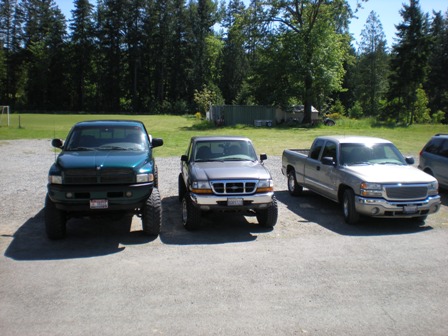The photograph shows three pickup trucks parked on a concrete parking lot without lines, accompanied by the partial view of a minivan on the far right. Positioned from left to right, the first truck is a glossy blue with prominent front-facing features such as large black wheels and visible headlights. Next to it is a tan or silver truck with orange and clear headlights and slightly green-tinted windows. On the right side, there's a slightly larger, shiny silver truck with black wheels, catching the sunlight intensely. All vehicles are arranged horizontally. Behind the trucks, there is a clear grassy area transitioning into a backdrop of tall trees with dense foliage, and a faint glimpse of a soccer goal is visible among the greenery. The scene is set under a bright, clear sky, enhancing the overall vividness of the day.